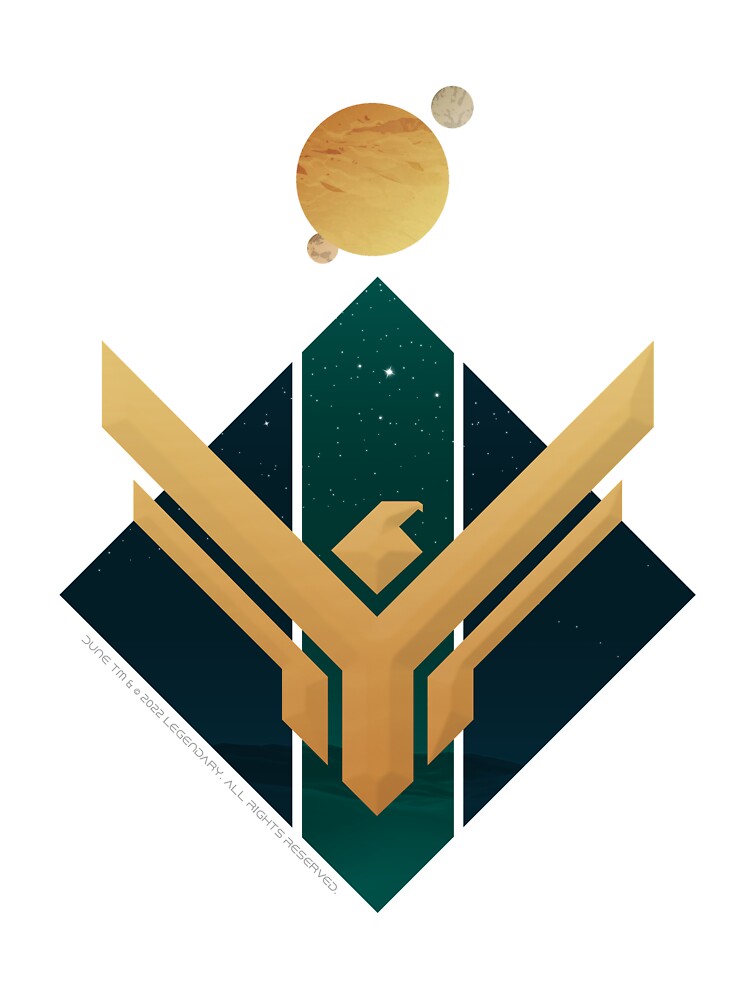The image features a white background with a prominent design. Near the top is a large, light brownish-orange circle, resembling a planet, with some darker patches. Surrounding it are two smaller circles, one in the top-right and the other in the bottom-left. Below these circles is a diamond-shaped figure tilted on its side, with a solid green stripe running vertically in the center, flanked by dark triangles divided by white lines. Tiny white stars are scattered within the green stripe and triangles. Superimposed on the diamond shape is a stylized golden eagle, composed of geometric shapes, with a head resembling an eagle perched at the top and extending L-shaped wings. There's small, barely legible text along the bottom left corner that includes "Dune TM copyright 2022 legendary all rights reserved," indicating a possible connection to the movie "Dune."